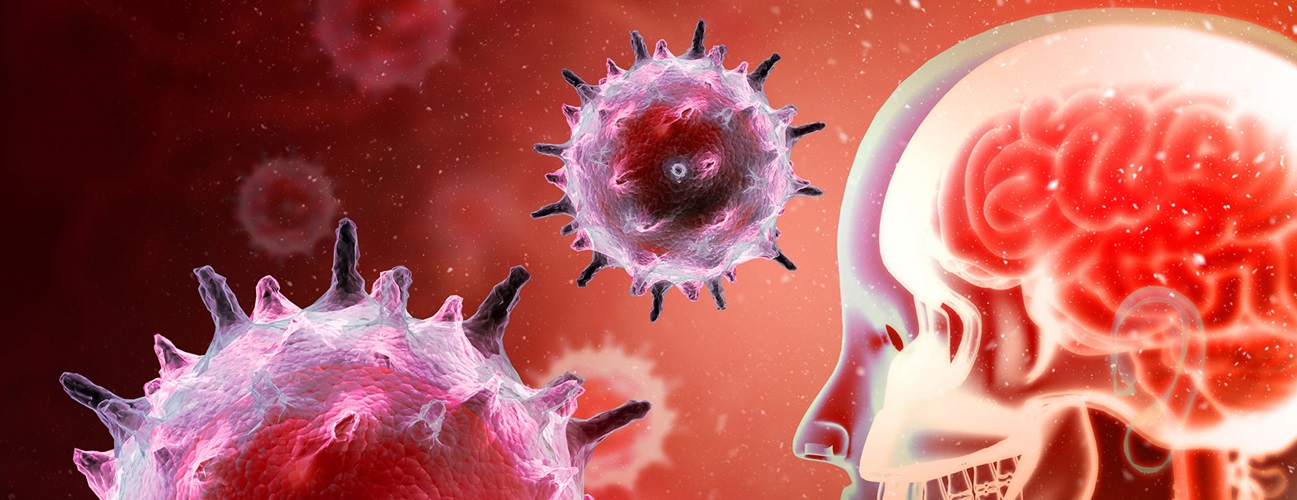This is a computer-generated illustration featuring a detailed cross-section of a human head. The transparent layers reveal the skull, depicted in lavender, and the brain, colored in dull red. The background is predominantly reddish, providing a stark contrast to the intricate details inside the head, which also include the teeth, ear, and the beginning of the spine. Floating around the head are spherical virus-like objects, resembling COVID-19 with their spiky surfaces. These spheres are rendered in hues of magenta, red, pink, and purple, giving a surreal and somewhat menacing touch as they appear to be targeting the brain and face. The artistic style combines realism with an abstract, almost animated quality, making the image visually striking and evocative.